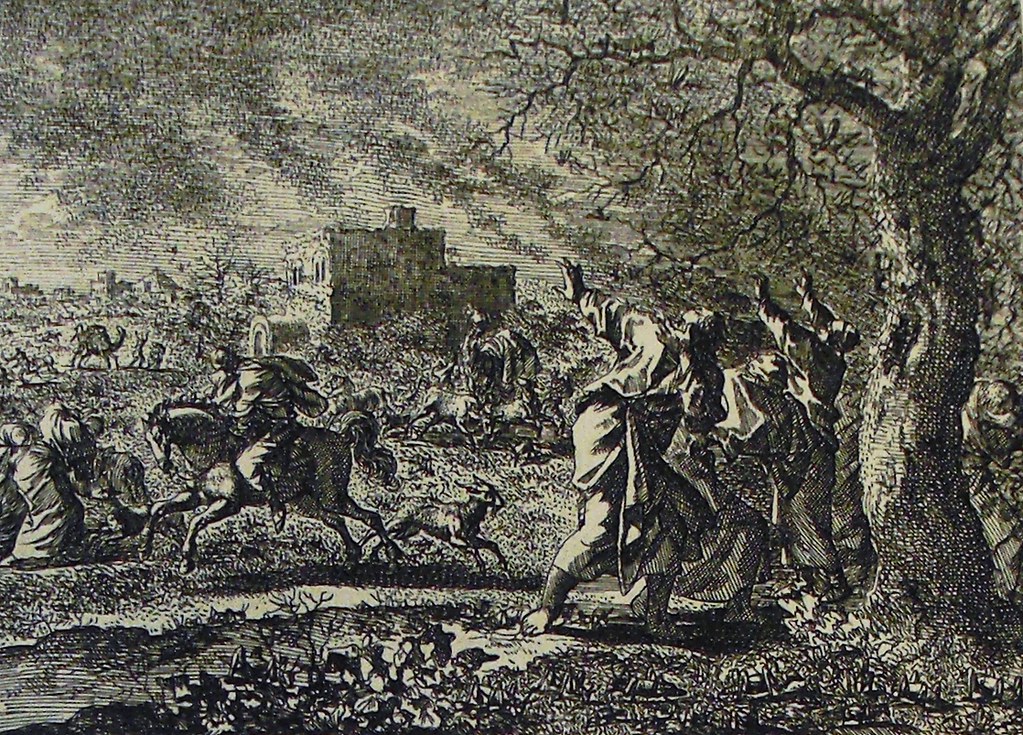The painting, rendered in a striking monochromatic palette, captures a series of evocative scenes seamlessly intertwined. On the right side, a striking tree stands tall, its branches stark against the background. Spread throughout the composition are several figures donned in flowing dresses, with some raising their hands skyward in expressive gestures. Three distinct individuals are particularly noticeable, their hands lifted as if in a moment of epiphany or appeal.

In the center of the painting, a dog sprints to the right, its motion contrasting with the static elegance of a man on horseback, who trots to the left, providing a dynamic juxtaposition. Nearby, a figure appears engaged in a task, possibly aiding a camel by securing a bag onto its back, indicating a scene of travel or trade.

A prominent building with four defined corners anchors the far center of the painting, adding an element of structure and stability to the otherwise fluid and narrative-rich landscape. The ground beneath these various scenes is rendered in darker shades, providing depth and grounding to the illustration, while the sky above is painted in lighter tones, offering a brilliant contrast that accentuates the subjects below. This intricate and layered composition is a testament to the artist's ability to weave multiple stories within a single frame.